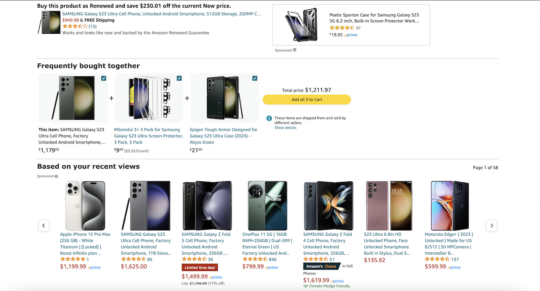**Detailed Caption:**

This image showcases an e-commerce website displaying a vertically long, white webpage structured into three distinct sections delineated by gray or black lines.

**Top Section:**
On the left side at the top, there's a promotional offer indicating discounts for purchasing a renewed product. The text mentions potential savings of up to $230.01 off the current new price. Below this, an image of a Samsung Galaxy S23 Ultra cell phone is visible, alongside additional information about shipping and product ratings, which indicate the phone has garnered four and a half stars based on several customer reviews. Adjacent to this information, similar details are provided for a different phone model.

**Middle Section - Frequently Bought Together:**
The middle section titled "Frequently Bought Together" similarly displays a Samsung Galaxy S20 (or possibly another model such as S23 or S29), priced at approximately $1,179.00. It shows a combination of this phone with two other products, which appear to be accessories like a cover. This section includes a button labeled "Add All Three to Cart," with the cumulative price of $1,211.97 shown in green boxes with white check marks, indicating that these items have been selected.

**Bottom Section - Based on Your Recent Reviews:**
The final section, titled "Based on Your Recent Reviews," presents a carousel of approximately seven phones, with prices ranging from $1,625.00 to $135.92. These phone options are arranged horizontally, providing a comprehensive display of various models recommended to the user based on their browsing history.

Overall, the image depicts a streamlined e-commerce interface guiding the user through product offerings, bundled recommendations, and personalized suggestions.